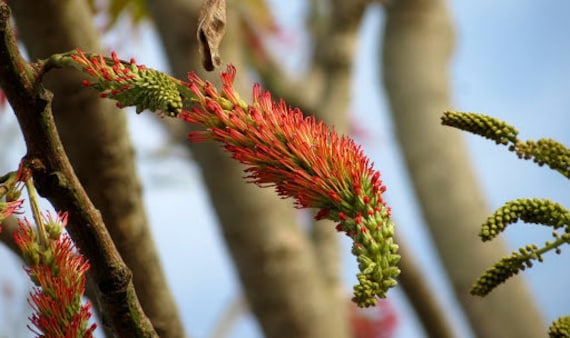This horizontal rectangular photograph captures the intricate beauty of an unusual flowering bush or tree with thick, smooth stems. Dominating the foreground, a unique flower emerges with green-tipped buds that transition into striking red, hair-like threads as they bloom. The contrasting textures and colors suggest a delicate transformation from the seedy green top to the vibrant red bloom. 

Centered in the image, a partially bloomed flower showcases this vivid transition, while to its right, a cluster of mostly red flowers adds a splash of color. On the left side, a trio of green buds awaits their full blossoming. The stems, adorned with these flowers, are attached to a larger, out-of-focus tree with a thicker trunk positioned in the background. 

Framed against a clear blue sky with hints of white clouds, the composition highlights both the intricate details of the flower and the larger, smooth woody elements of the plant. The sensory contrast between the smoothly textured stems and the delicate, thread-like blooms accentuates the plant's unique structure and adds depth to the image.